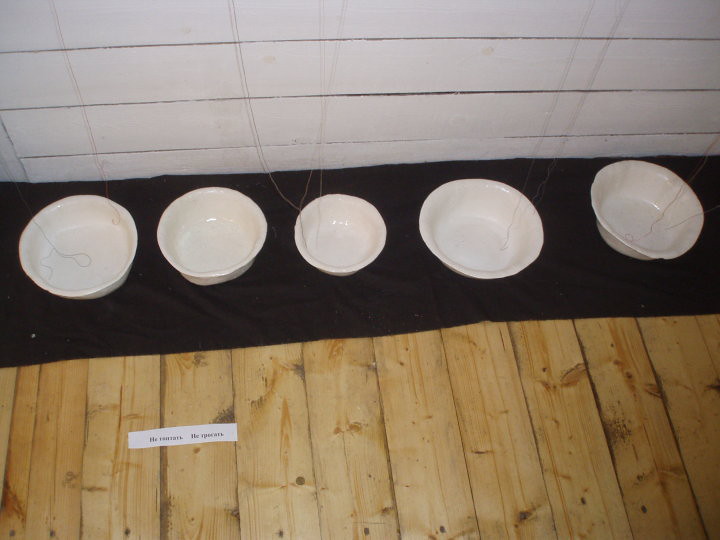This photograph captures a meticulously arranged scene featuring five white ceramic bowls lined up on a long, rectangular black cloth. The setup is situated on a vertically slatted wooden floor, showcasing a natural wood finish. Behind the bowls is a white wall with horizontal wooden slats. The bowls, varying in size with the central one being noticeably smaller, appear slightly misshapen, hinting at an imperfect crafting process. Some strings can be seen emerging and dangling into a couple of these bowls, adding an additional layer of curiosity. Towards the lower left corner of the scene, a long, skinny piece of paper with unreadable text is placed on the floor, further contributing to the enigmatic nature of the photograph.